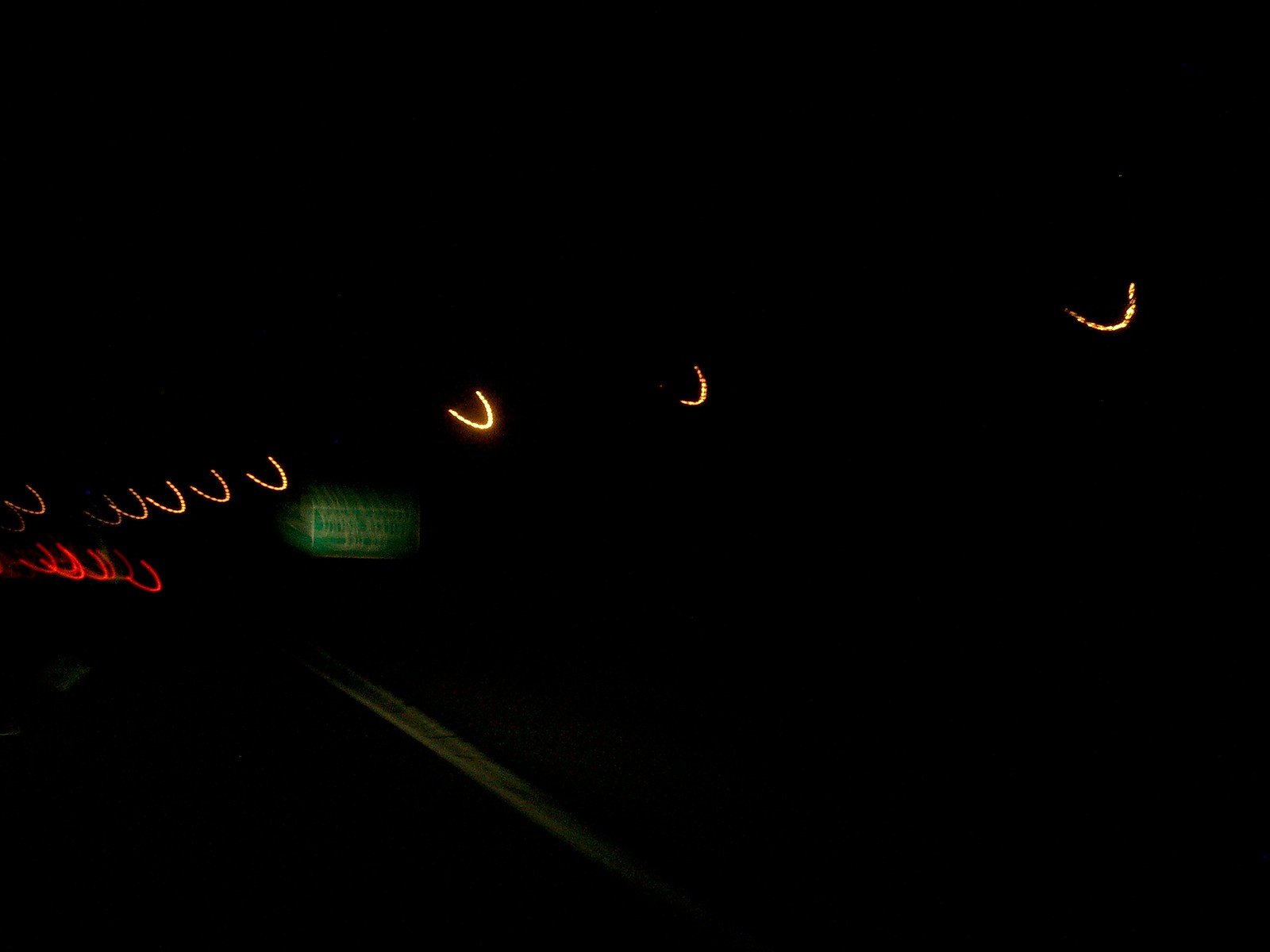The image depicts a dark, blurry nighttime highway scene, with an otherworldly, almost surreal atmosphere characterized by heavy, sleepy eyes. The road appears shadowy, defined only by faint reflective paint marking lane boundaries. Yellow and white lights, along with scattered U-shaped red lights, punctuate the darkness. A green rectangular highway sign is discernible, though its text is unreadable due to the photo’s blurriness. Despite the pervasive blackness, the V-shaped lights floating in the air add to the eerie glow, vaguely illuminating the scene. The car emitting light onto the road is not visible, but its effect on the scene is apparent. The image captures a sense of driving through an obscured, nocturnal landscape where clear details are swallowed by the night.